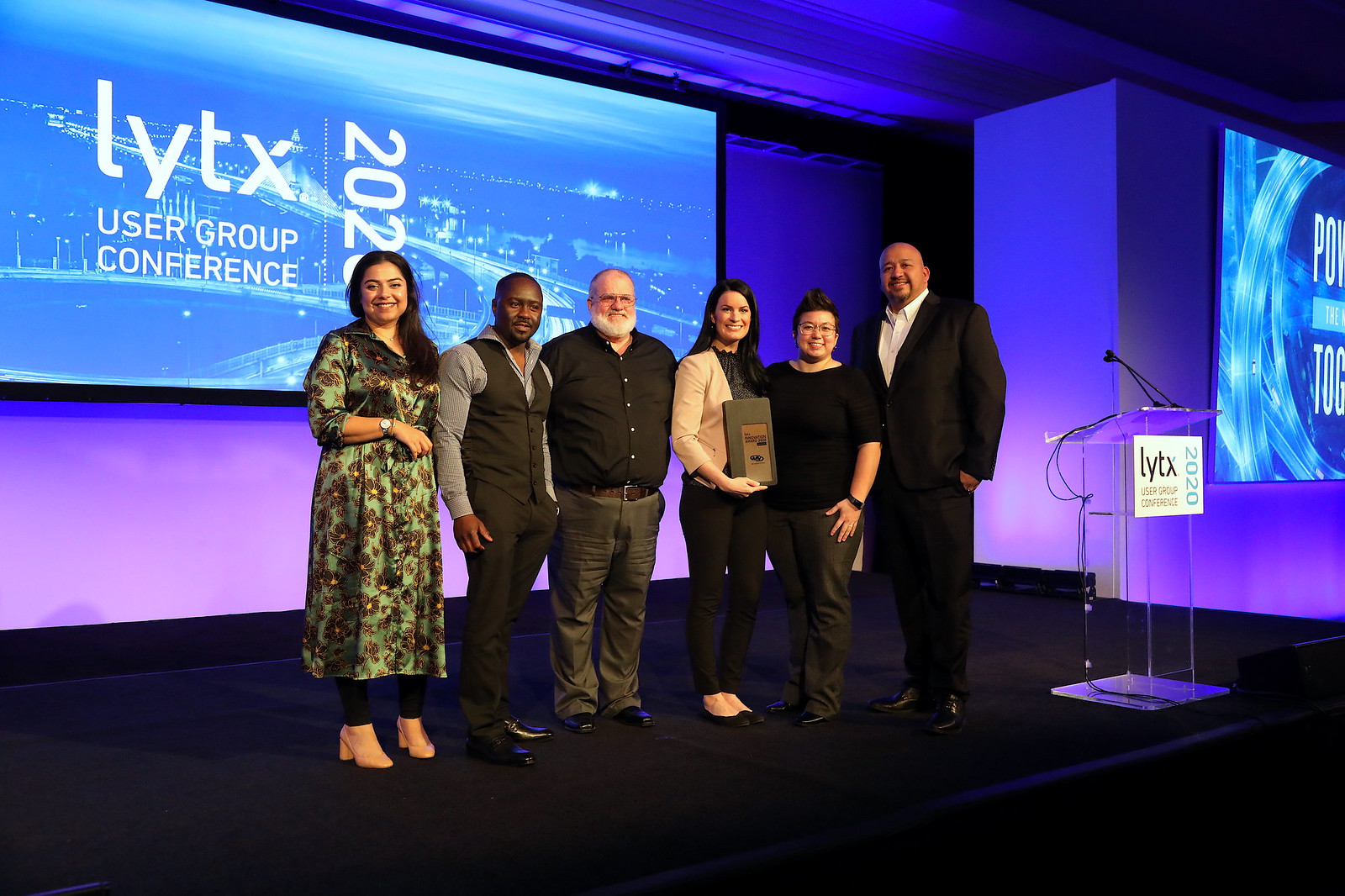A photograph captures a group of six individuals, three men and three women, standing on a stage and smiling at the camera. The woman at the center proudly holds a small, brown award, her achievement clearly a focal point of the scene. The stage is bathed in blue light, with blue walls enhancing the backdrop. Behind the group, a large screen displays a cityscape with white text reading, "Lit X User Group Conference 2020." The joyous expressions on their faces suggest a moment of triumph and celebration.